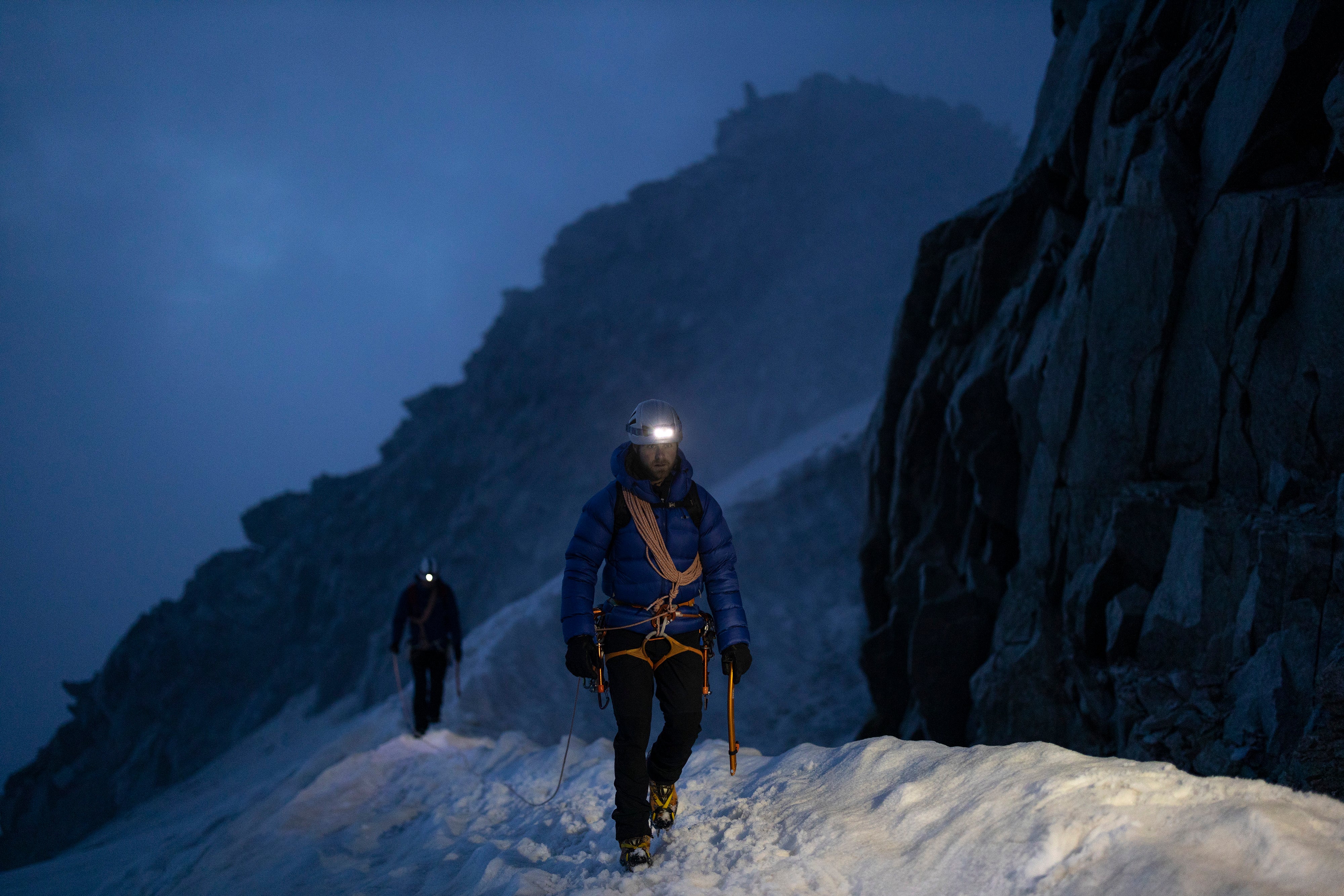The image depicts two mountain climbers navigating a snowy mountain slope at night. Both climbers are equipped with helmets that have lights, illuminating their path as they descend to seek shelter before more snowfall occurs. They are dressed in thick jackets, suitable for the frigid conditions, with the first climber wearing a dark blue jacket and orange ropes around his neck. The setting is a mountainous area, characterized by extensive snow and a gray, cloud-covered sky, suggesting minimal sunlight or nighttime. The climbers are connected by a rope, emphasizing their need to stay close together for safety. The terrain is described as relatively flat where they are walking, but the mountain slopes can be seen in the background. The photo's color scheme includes white, orange, blue, and some brownish hues, highlighting the stark, cold environment of the frozen tundra they are traversing.